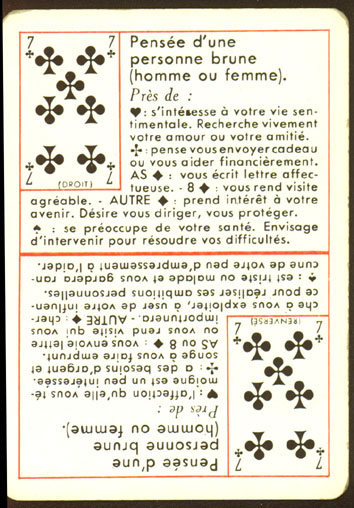The image depicts an aged, cream-colored playing card with a yellowish tint, suggesting its vintage nature. The card is centered against a black background with a thin black border. Notably, the card features two distinct horizontal red rectangles, providing information on a game in French. 

In the upper red rectangle, a large, prominent seven of clubs symbol is positioned in the top left corner. Next to this symbol, a block of French text is displayed in large letters, followed by a couple of paragraphs in smaller French text providing detailed instructions.

Mirroring the top half, the bottom red rectangle replicates the same seven of clubs symbol, text in large letters, and instructional paragraphs. However, this section is inverted, with the seven of clubs in the bottom right corner and the text appearing upside down and reversed, creating a symmetrical design with the top half.

The card’s edges show signs of wear, with slightly blackened and folded corners, enhancing its antique appearance.